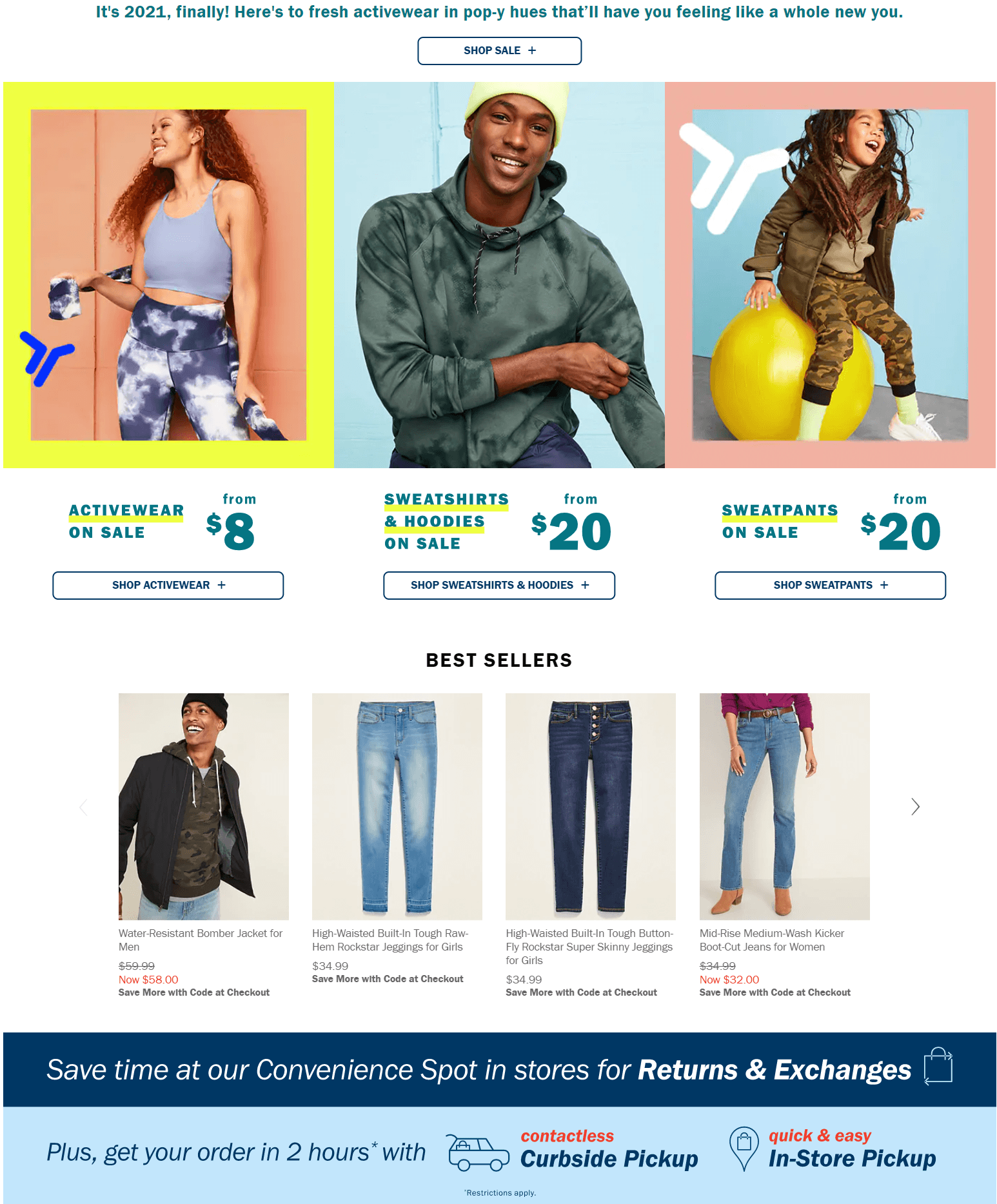The website interface displays a prominent header celebrating the arrival of 2021 with a message encouraging users to embrace a new start with fresh activewear and vibrant hues. A "Shop Sale" button is placed immediately below the message, inviting visitors to explore current promotions.

Beneath the header, three images are displayed in a row, showcasing various product categories. Following this, a "Bestsellers" section features a row of four images, each highlighting popular items.

1. **First Image (Left)**
   - **Border:** Yellow
   - **Text:** "Activewear on sale from $8"
   - **Button:** "Shop Activewear"
   - **Subject:** A woman dressed in gym wear, possibly for yoga.

2. **Second Image (Center)**
   - **Text:** "Sweatshirts & Hoodies on sale from $20"
   - **Button:** "Shop Sweatshirts & Hoodies"
   - **Subject:** A man wearing a hoodie.

3. **Third Image (Right)**
   - **Text:** "Sweatpants on sale from $20"
   - **Button:** "Shop Sweatpants"
   - **Subject:** A child with long dreadlocks dressed in sweatpants.

The "Bestsellers" section includes detailed product listings: 

1. **Men’s Water-Resistant Bomber Jacket**
   - **Price:** Originally $59.99, now $58.
   
2. **Girls' High-Waisted Built-In Tough Rockstar Legging Jeggings**
   - **Price:** $39.99 
   - **Offer:** Save more with a promo code at checkout.

Each image and description is optimally placed to attract customers by highlighting the discounts and various trendy clothing options available.